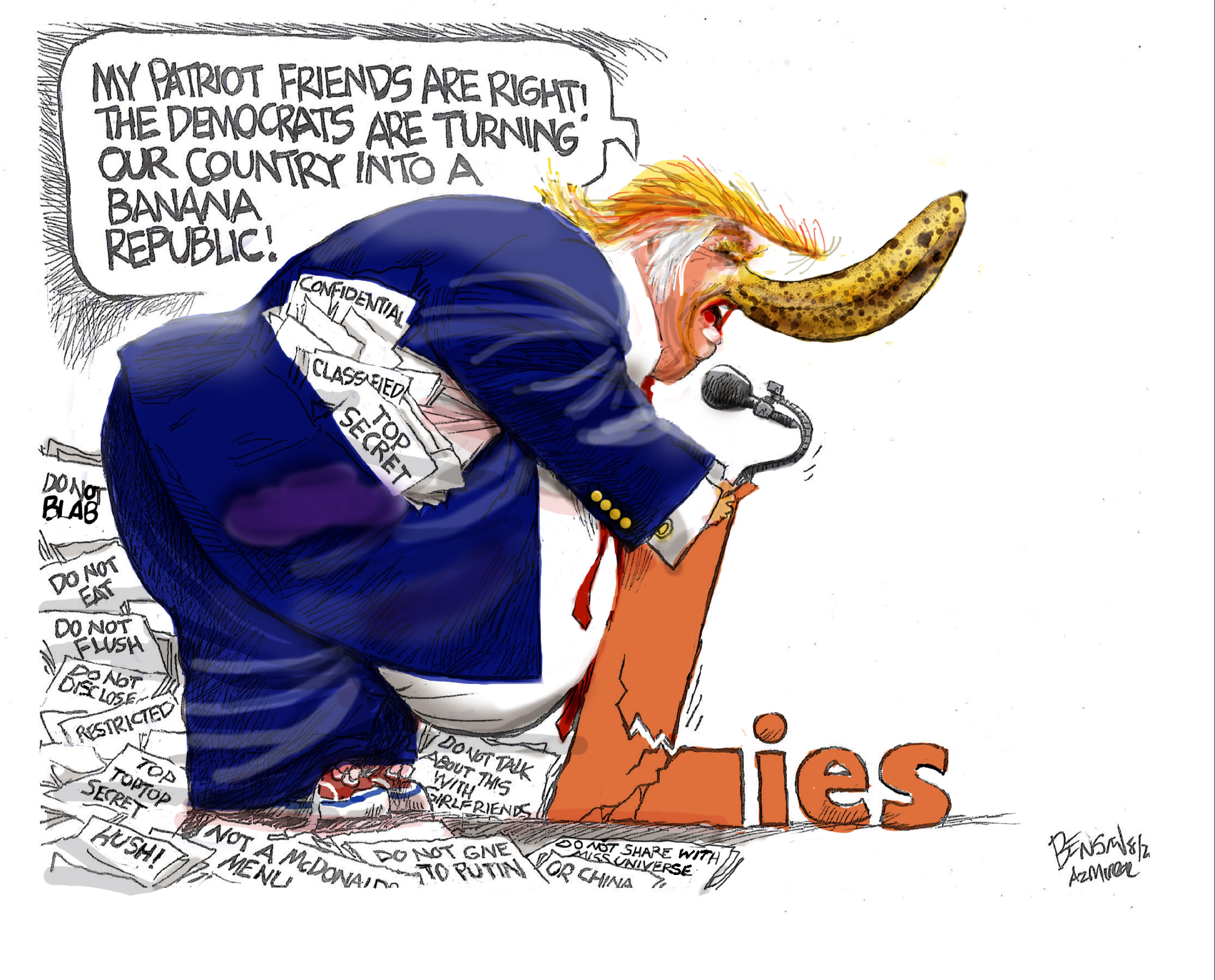This is a square-cropped political satire cartoon, seemingly taken from a newspaper and signed by the artist in the bottom right corner as "Ben, SML 82, AZ." The cartoon depicts a grotesquely obese former President Trump with yellowish hair and white sideburns. His stomach protrudes outward in a circular shape, cracking the lectern beneath him. Trump is leaning over and shouting into a microphone attached to a large, cracked letter "L" that spells out "lies," with the "IES" portion lying horizontally at the bottom in smaller letters. His nose is humorously drawn as a decaying banana, complete with brown spots. He wears a blue suit with gold buttons on the sleeves and is surrounded by confidential documents, some of which are spilling onto the floor. In the upper left corner, a thought bubble reads, "My patriot friends are right. The Democrats are turning our country into a banana republic." There are also some newspapers with headlines scattered beneath the text bubble.